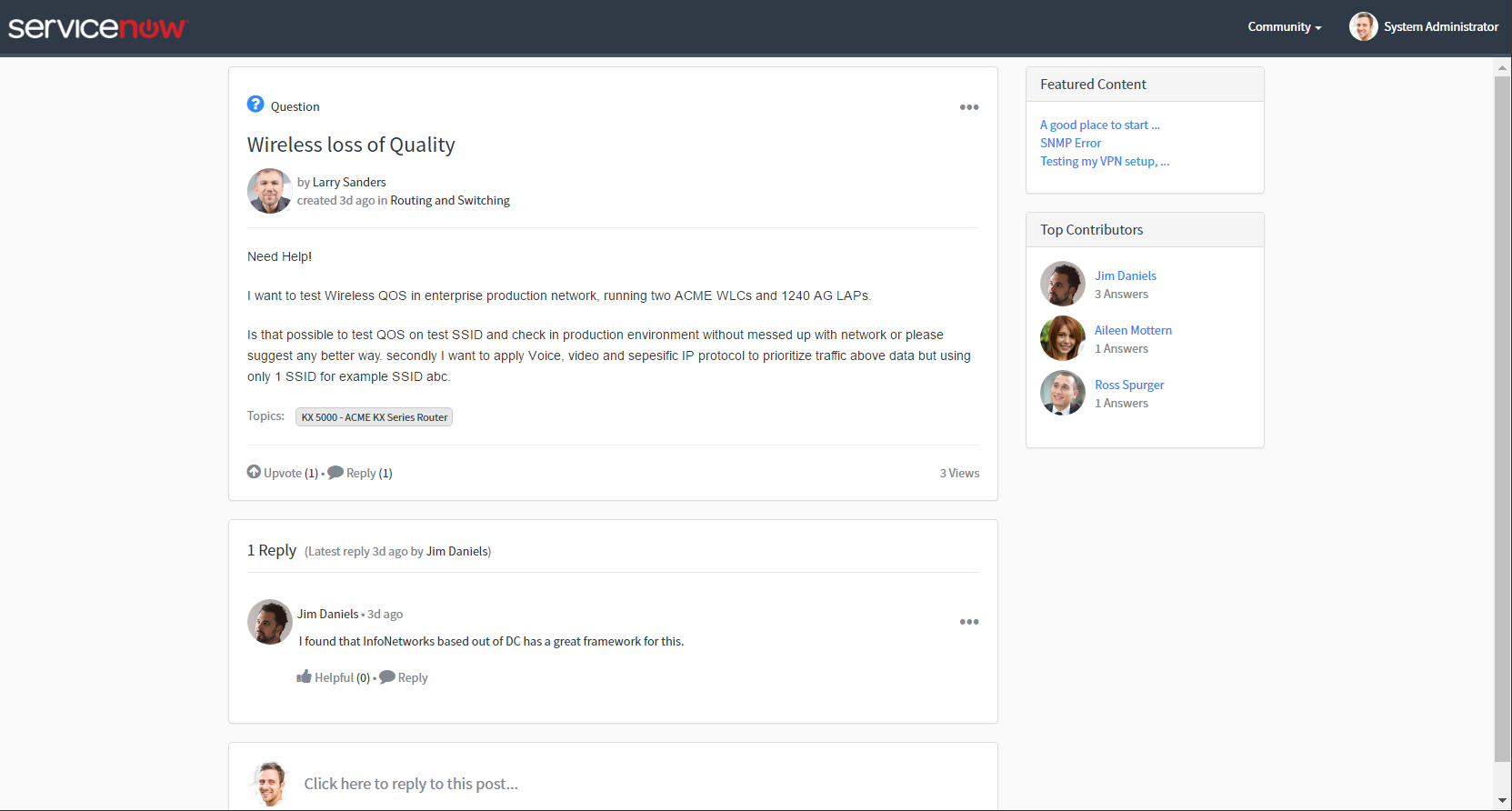At the top of the website, there is a black border. On the upper left-hand side, the word "Service" is displayed in white text next to the word "Now" in red text. On the upper right-hand side, "Community" is written in white text accompanied by a downward-pointing arrow. Below it, the page displays the text "System Administrator" next to an image of a person.

The overall background of the page is off-white, while specific sections feature white boxes. The foremost white box contains several pieces of information:

1. **Question Title:** "Wireless Loss of Quality" by Larry Sanders
2. **Created:** Three days ago
3. **Category:** Routing and Switching

The main content of the query reads: "Need help? I want to test wireless QoS in an enterprise production network running two ACME WLCs and 1240 AGL APs. Is it possible to test this on the SSID and check it in a production environment without disrupting the network? Or could you please suggest a better way? Secondly, I want to apply a voice and video-specific IP protocol to prioritize traffic above data using just one SSID, for example, SSID ABC."

One person, Jim Daniels, responded three days ago. His reply, highlighted in black text, states: "I found that Info Networks, based out of D.C., has a great framework for this." 

Below the response, there are options to mark the reply as "Helpful" or to submit a follow-up reply.